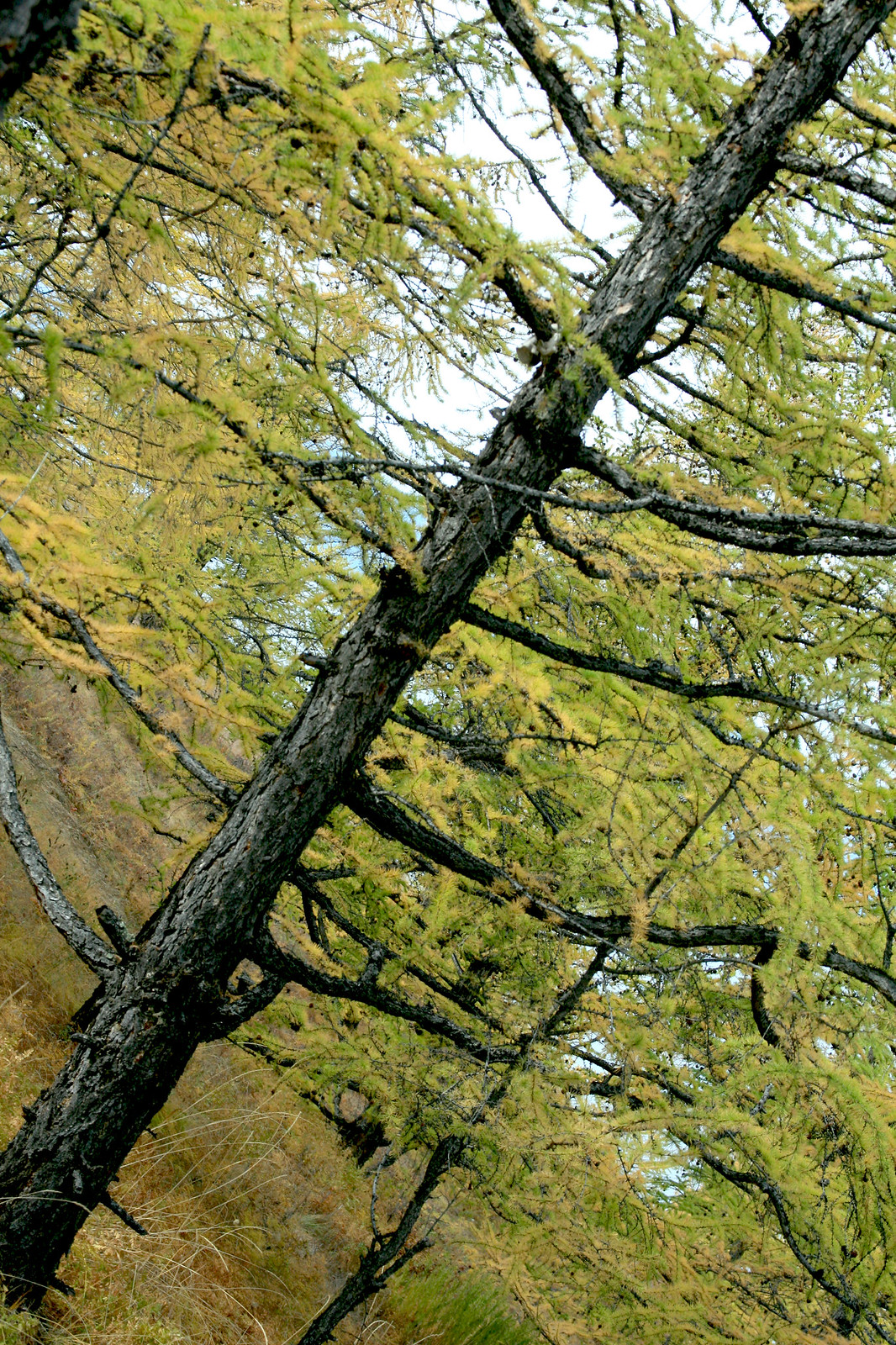This is a detailed image of a tall, prominent tree captured outdoors during the daytime. The tree's dark, thick trunk emerges diagonally from the lower left corner of the photograph, extending to the upper right corner. It's framed by a forest environment with a lush, green backdrop of grasses, bushes, and other trees. While the tree's branches and leaves mainly fill the right side of the image, a smaller tree can also be seen nearby. The leaves on the tree are predominantly green, suggesting spring or early autumn, and while some light filters through, the foliage largely obscures the sky. The overall photograph resembles the dimensions of a magazine page, emphasizing the natural beauty of this tranquil, wooded area.